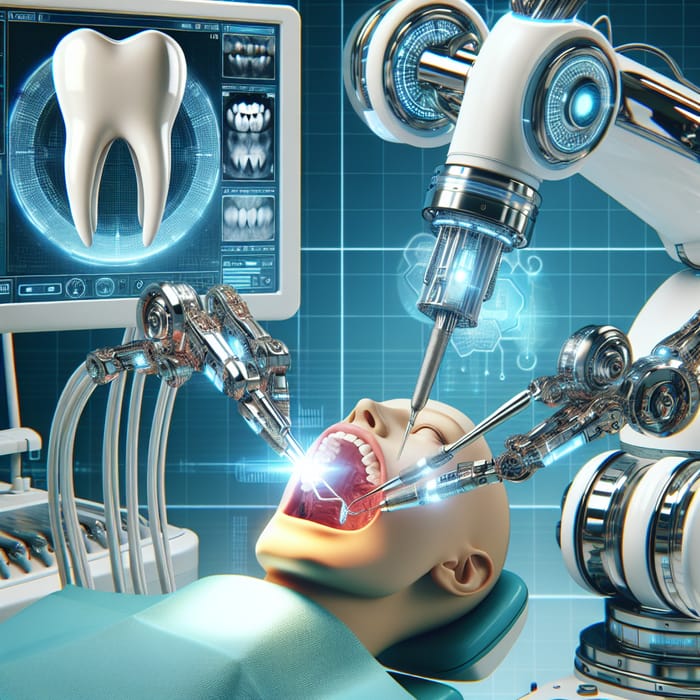The image is a detailed computer-generated graphic depicting a futuristic dental procedure. A bald person, possibly Caucasian, is laying back in a dentist's chair with their mouth wide open, exposing their teeth all the way to the molars. Above their head, an intricate array of robotic tools and machinery operate. One prominent arm, located at the top right, has a white body with blue shiny lights and extends downward with a needle-like attachment at its tip. Another arm features two wheels at its elbow, bending forward to hold a small mirror and what looks like a washing machine component, aiding the procedure.

From the left side, a spray tube, resembling typical dentist equipment, connects to a machine that casts a shiny light on the person’s teeth. The graphical representation includes exaggeratedly peeled back lips and highly visible roots, lending an almost surreal quality.

In the background, a large vertical monitor displays a comprehensive view of the ongoing dental work, including a detailed image of a white molar and x-rays of the individual’s teeth. The entire scene, captured in a rectangular photo, captures the advanced, almost sci-fi atmosphere of the setting.